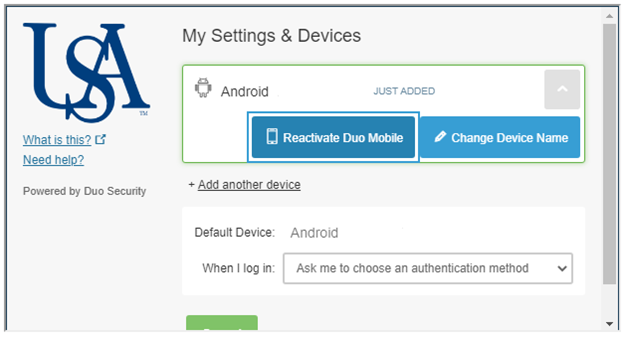This image is a detailed screenshot that is enclosed within a light gray, thin-line border on the left, top, and right sides. The upper left corner of the screenshot prominently features a bold blue logo with the letters "USA," where the U and A are connected, and the S sits atop both letters. Directly beneath the logo, in blue text, are the links “What is this” and “Need help.” Below these links, there is a note indicating that the service is "powered by Duo Security."

To the right of the USA logo, the heading “My Settings and Devices” is displayed. Under this heading, there are two buttons. The first button is labeled “Reactivate Duo Mobile,” which is highlighted in blue, and the second button is labeled “Change Device Name” with a small pencil icon to the left of the text, indicating an option to edit.

In the upper left corner of the main section of the screenshot, the term "Android" is indicated, suggesting the operating system relevant to the settings shown. Below that, there is an option labeled “Add another device,” followed by “Default Device.” Next to “When I log in,” there is a pull-down menu that states “ask me to choose an authentication method,” offering the user choices for their preferred security authentication steps during login.